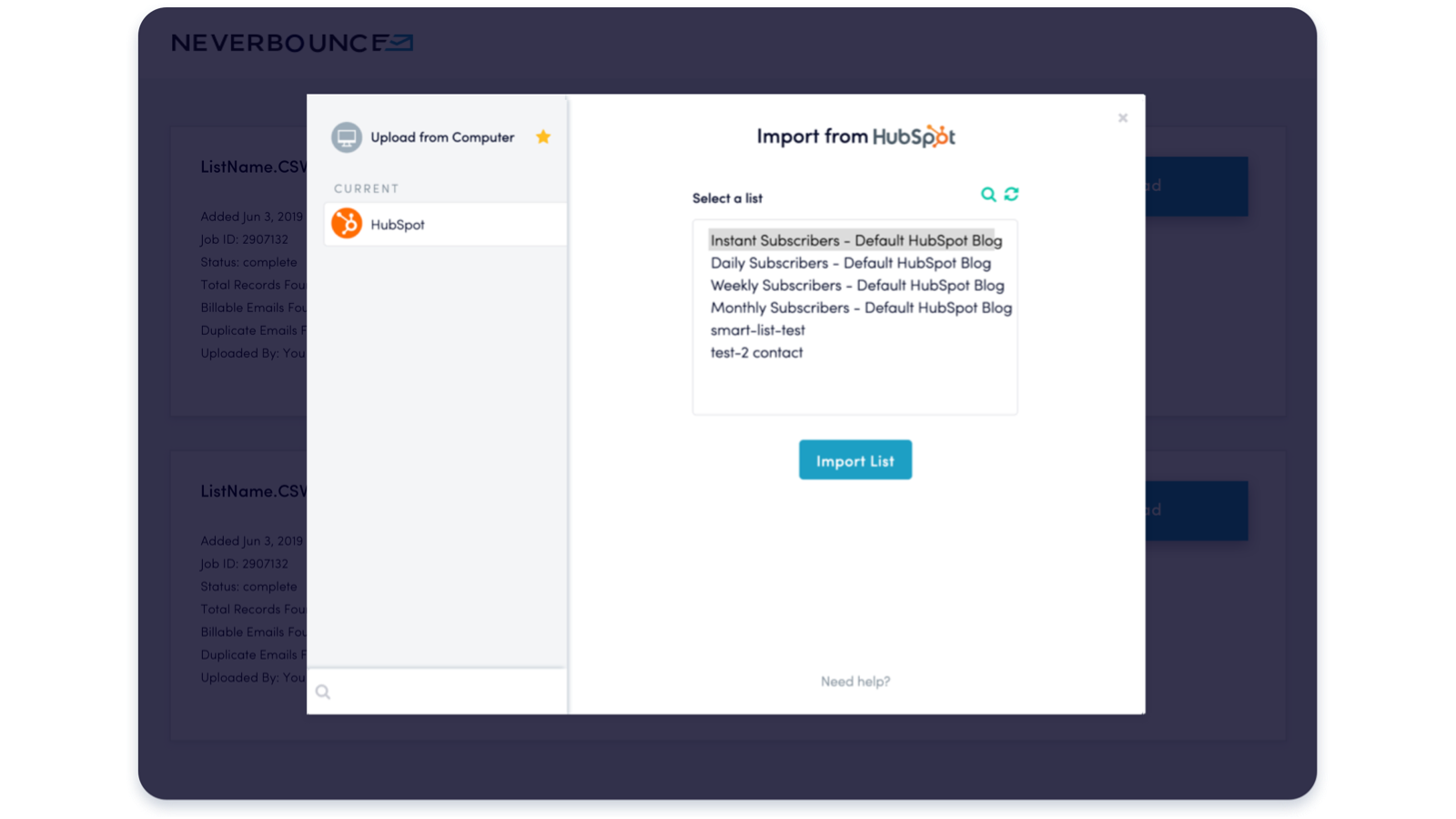A small, low-resolution image depicts a gray-tinted webpage identified as "Never Bounce" in the top left corner, accompanied by a logo and several icons. Directly below, there are two white boxes containing black text headers and paragraphs. On the right side of the screen, a blue rectangular button is visible. Centrally, a pop-up box dominates the image, featuring a gray circle in the top left, next to the text "Upload from Computer." Adjacent to these elements is a gold star, followed by an orange circle with text beneath it, and nearby, the words "Import from HubSpot" with additional text below. A blue hyperlink and several lines of smaller text are present within this pop-up. At the bottom of the pop-up, a blue rectangular button with white text stands out. The very bottom of the image contains text that is illegible.